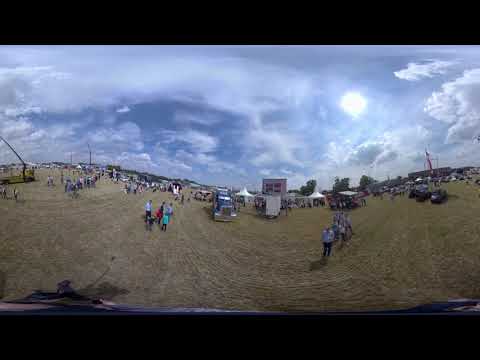This photograph depicts a bustling outdoor festival or carnival taking place on a large open field covered with green grass, though some areas show dirt track marks from vehicles. The image has been captured with a fisheye lens, curving the surrounding sky and ground into a concave form. The sky is a mix of blue and white clouds, with the sun shining brightly in the top right corner. Numerous people have gathered on the field, where makeshift shops and various types of tents are set up amidst parked cars and trucks. Notable elements include a fire truck with an extended basket on the left side and a blue 18-wheeler cab centrally positioned, facing slightly to the right, near tents of various colors and sizes. A pinkish two-story building with central windows is visible to the right of the truck, followed by more tents and parked cars further to the right. The scene is lively, with groups of people enjoying what appears to be a sunny yet cloudy day, and American flags fluttering in the air. The curvature from the fisheye effect is accentuated by horizontal black strips on the top and bottom of the image, framing the vibrant activity.